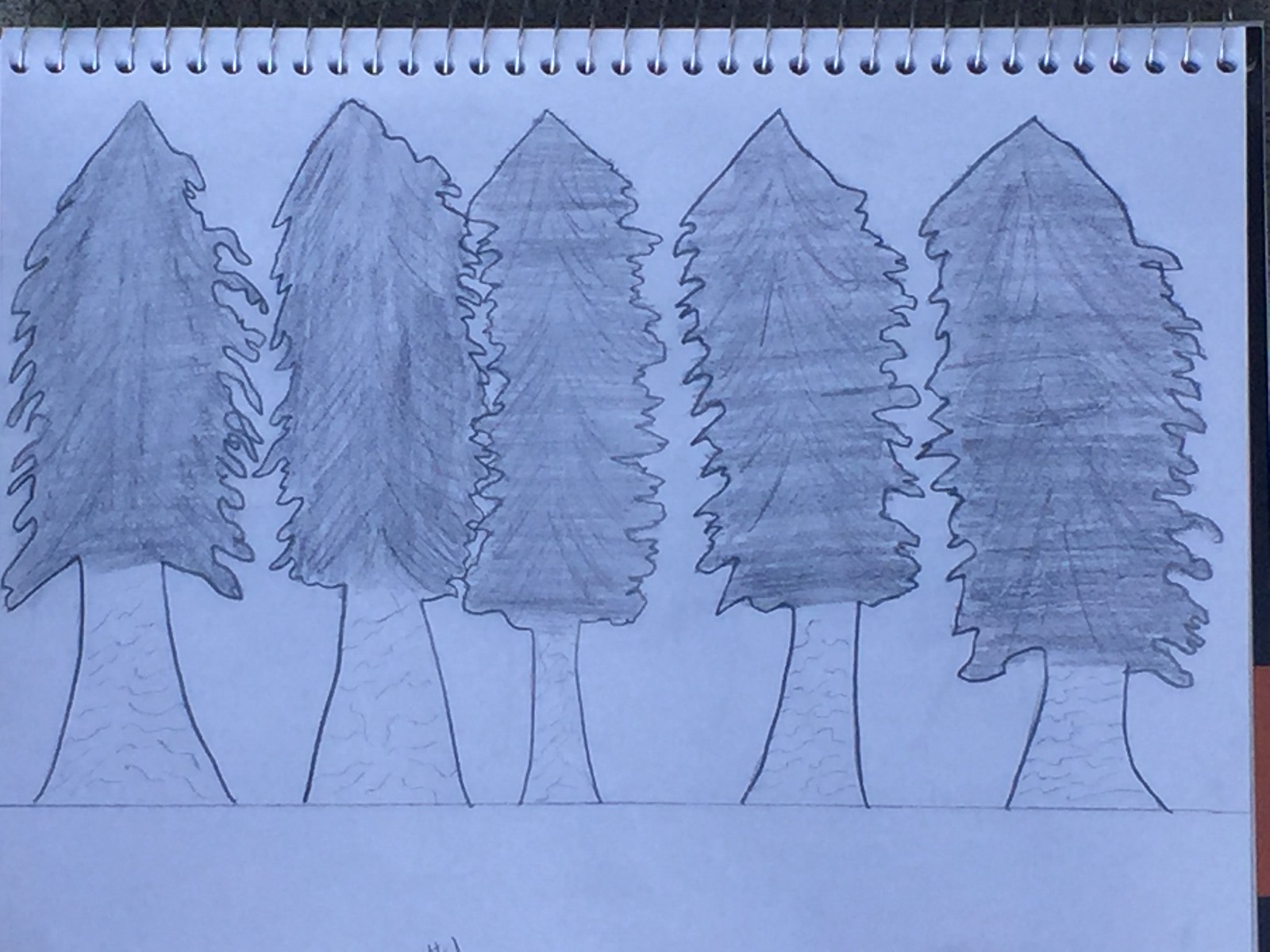This image features a detailed sketch of five unique trees drawn on a sheet of flat white paper within a silver-looped spiral notebook. The paper is unlined, resembling copy paper rather than conventional notebook paper. The trees are meticulously sketched with pencil, each uniquely shaped yet collectively curving inward. The trunks are drawn with an emphasis on texture and detail resembling bark patterns, appearing mostly white with some sketch lines giving depth. The base of the first tree is wider and gradually narrows towards the top, featuring a serrated edge. The two leftmost trees are slightly wider and have a less sharp appearance compared to the others. A straight horizontal line at the bottom of the page represents the ground, grounding the drawing. The background remains plain, allowing the intricately detailed trees to stand out prominently.